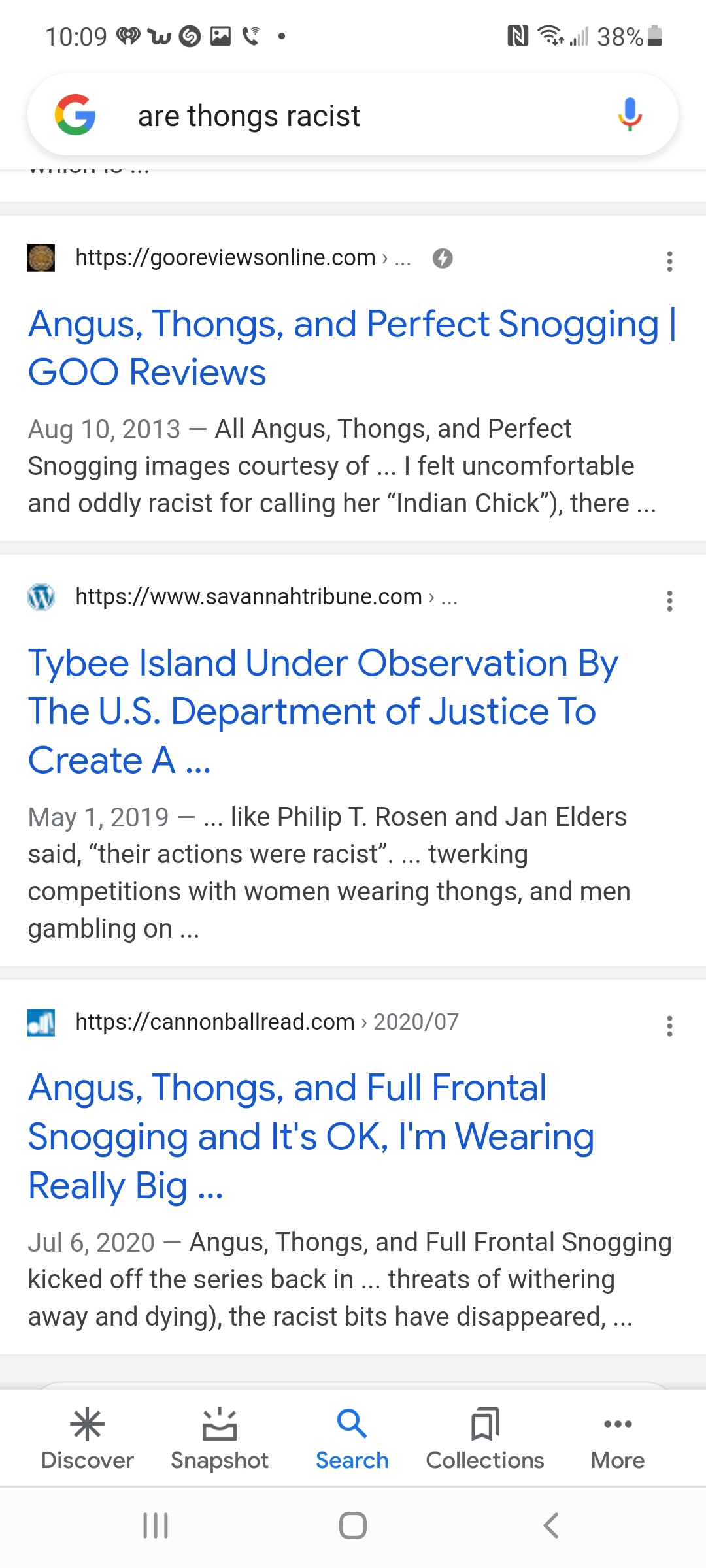The image depicts a screenshot from an Android phone displaying the Google app. The user has performed a search query asking, "Are thongs racist?" Scrolling down, three primary search result links are visible. 

The first link, labeled "Angus from Goo Reviews online," appears to reference "Angus, Thongs and Perfect Snogging" and includes images credited as "courtesy of." The visible text is cut off mid-sentence, ending with, "I felt uncomfortable in all the races for calling her 'Indian chick.'"

The second search result, from the Savannah Tribune, has a headline stating, "Tybee Island under observation by the US Department of Justice." A quote within this article mentions, "their actions were racist," followed by a description of "twerking competitions with women wearing thongs."

The final link, from cannonballread.com, seems to involve more content related to "Angus" and briefly mentions the word "racist," indicating the user has found articles associating the two terms.

At the bottom of the screen, navigation tabs are visible, including "Discover," "Snapshot," "Search," "Collections," and "More," with "Search" being active. The screen features a white background with blue links and black text for easy readability.